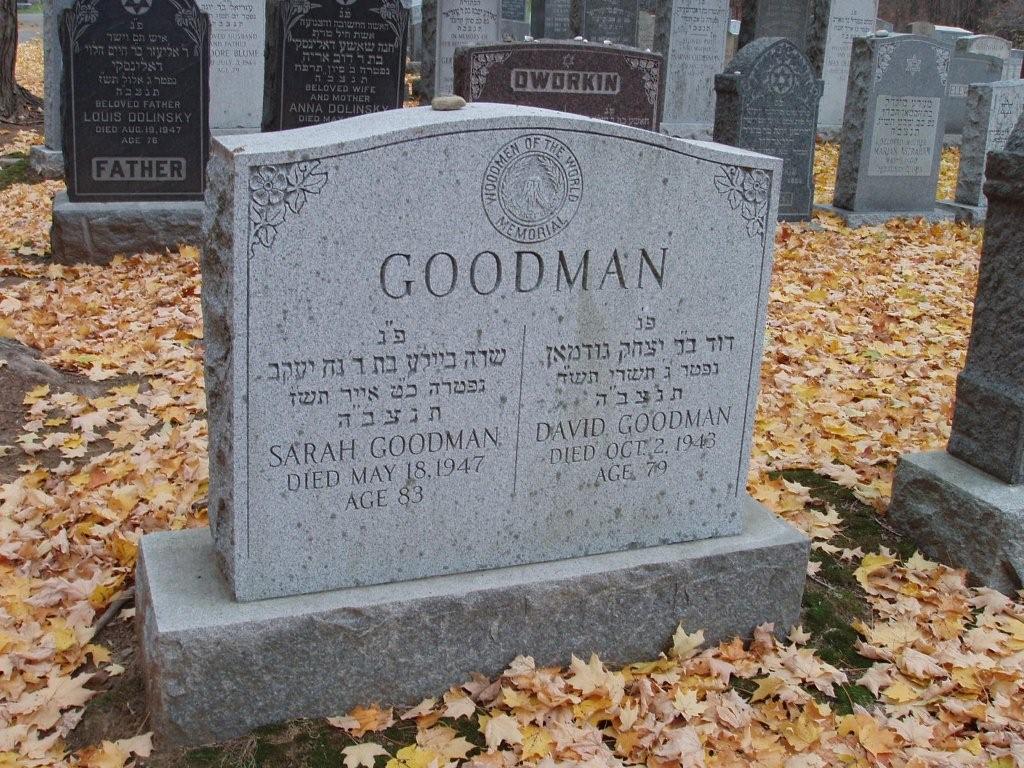This photograph captures an old, weathered headstone situated in a graveyard during the autumn season, as evidenced by the gold and beige leaves blanketing the ground. The headstone, crafted from gray stone with a curved, arched top and a carved circle at its center, prominently displays the surname "Goodman" above inscriptions mostly written in Hebrew. There are two distinct sections in the lower part of the headstone: on the left, it commemorates Sarah Goodman, who passed away on May 18, 1947, at the age of 83, while on the right, it honors David Goodman, who died on October 2, 1948, at the age of 79. A dividing line separates these two sections. In the background, numerous other gravestones are visible, creating a dense and solemn cemetery scene.